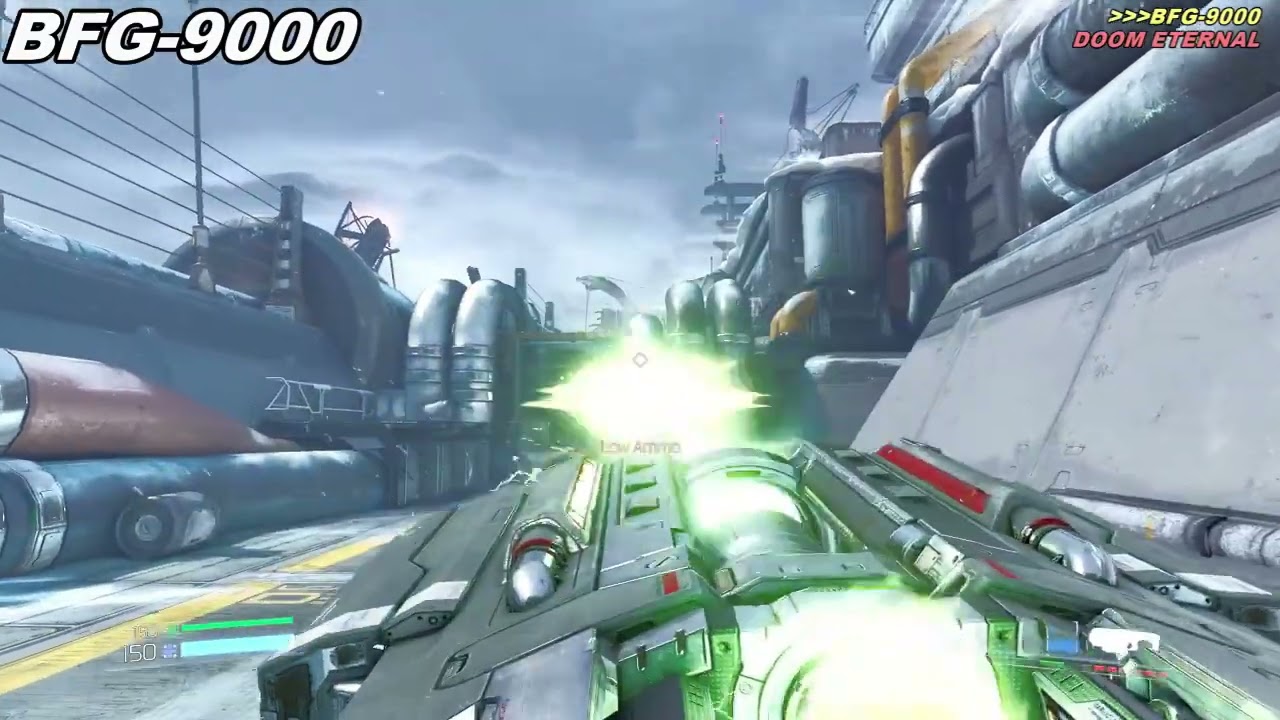In this detailed screenshot from the video game "Doom Eternal," prominently titled "BFG-9000" in bold white text at the top and subtitled "Doom Eternal" in yellow and red text on the right, we're looking at what appears to be an industrial, possibly sci-fi setting. Central to this image is a futuristic spaceship, gray with red trim and equipped with flaming engines at the back. This vessel has a distinctive lime green light emanating from its front, suggesting weapon fire. The scene is set against a backdrop of heavy, metallic machinery and industrial complexes on either side, reminiscent of an aircraft carrier deck or an advanced rail yard. The gray, cloudy atmosphere adds to the overall gritty, mechanical ambiance of the setting.